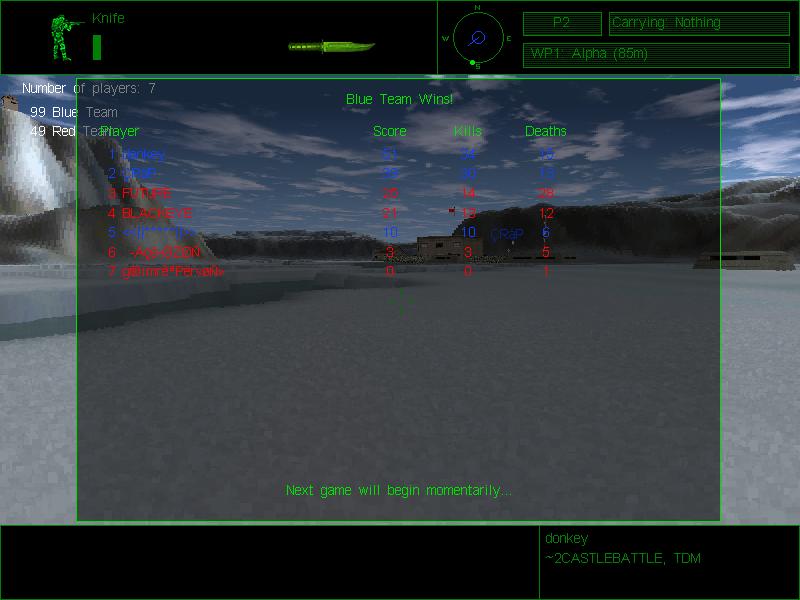This image is a screenshot of a computer game interface. The screen is bordered by black bars at the top and bottom. On the bottom black bar, the text "Donkey" is displayed on the right, followed by "Two Castle Battle, TDM" in green below it.

At the top black bar, the upper left corner features a figure holding a gun and wearing a backpack, highlighted in green. Next to this figure, the word "Knife" is displayed with a progress bar beneath it, and farther along the bar, there is a knife icon pointing to the right.

On the right half of the top screen, a compass (north, south, east, west) encircled is visible, with the label "P2" next to it. Below the compass, the text reads "Carrying Nothing," followed by "WP1 Alpha 85M" in parentheses, all in green.

Dominating the main screen is a semi-transparent box with the text "Next game will begin momentarily" at the bottom. At the top of this box, "Blue team wins" is declared, along with columns for "Player," "Score," "Kills," and "Deaths." 

In the background of the main screen, the image shows flat ground with hills or mountains in the distance, faintly visible through the semi-transparent elements. On the left-hand side, just below the top black bar, the number of players is listed as "Number of players: 7." Below this, the blue team’s score of "99" and the red team’s score of "49" are noted. 

The viewing box in front is overlaid but remains translucent, allowing the background scene to be slightly visible through it.